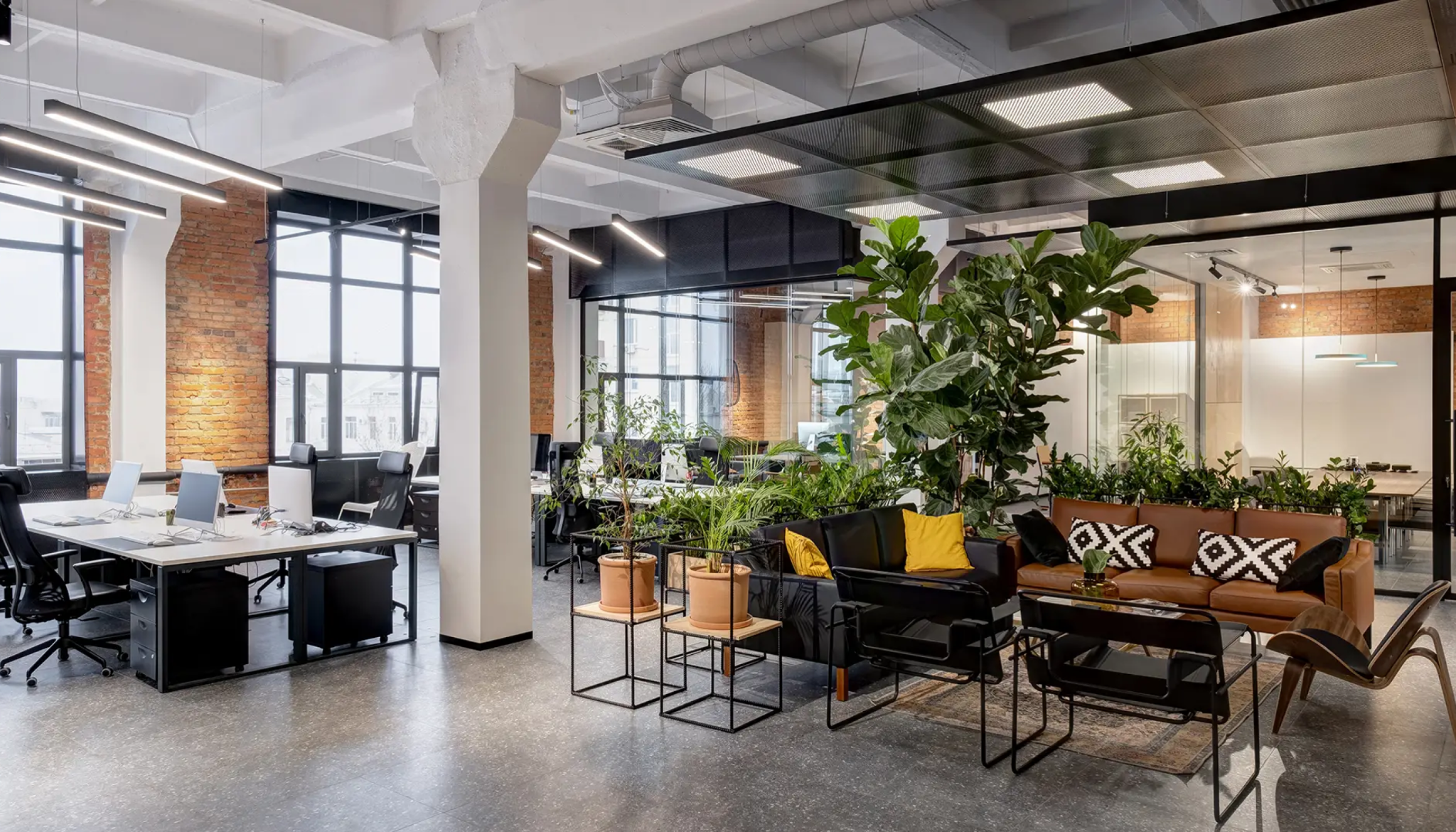The photograph showcases a meticulously designed and modernized co-working office space housed within a converted warehouse, retaining its industrial charm. The open-plan layout features exposed ductwork and tall beams, a testament to its original architecture. The ceiling has floating grids of black mesh with ceiling lights and dangling fluorescent shop lights, brightly illuminating various workstations and communal areas.

The left side of the image reveals expansive windows framed by exposed brick walls, allowing an abundance of natural light to pour in. Below these windows are desks designed to accommodate two to four workers, equipped with computer units and monitors. No people are present in the image, but the lights are on, giving an impression of readiness and modernity.

The seating area towards the center includes a black leather couch adorned with bright yellow throw pillows, a brown leather couch with additional throw pillows, and three contemporary chairs set around a rug. This inviting space is accentuated by a large potted ficus tree, ferns, and various other plants, adding a touch of natural greenery. Plant stands, made from a combination of wrought iron and wood, further enhance the aesthetic.

On the right side, solid glass walls partition smaller meeting rooms, maintaining the open and airy feel of the space. Polished cement floors add to its minimalist modern appeal, alongside squarish pillars supporting the overhead rafters. The overall color palette includes shades of white, gray, green, brown, and tan, contributing to a clean and serene work environment.